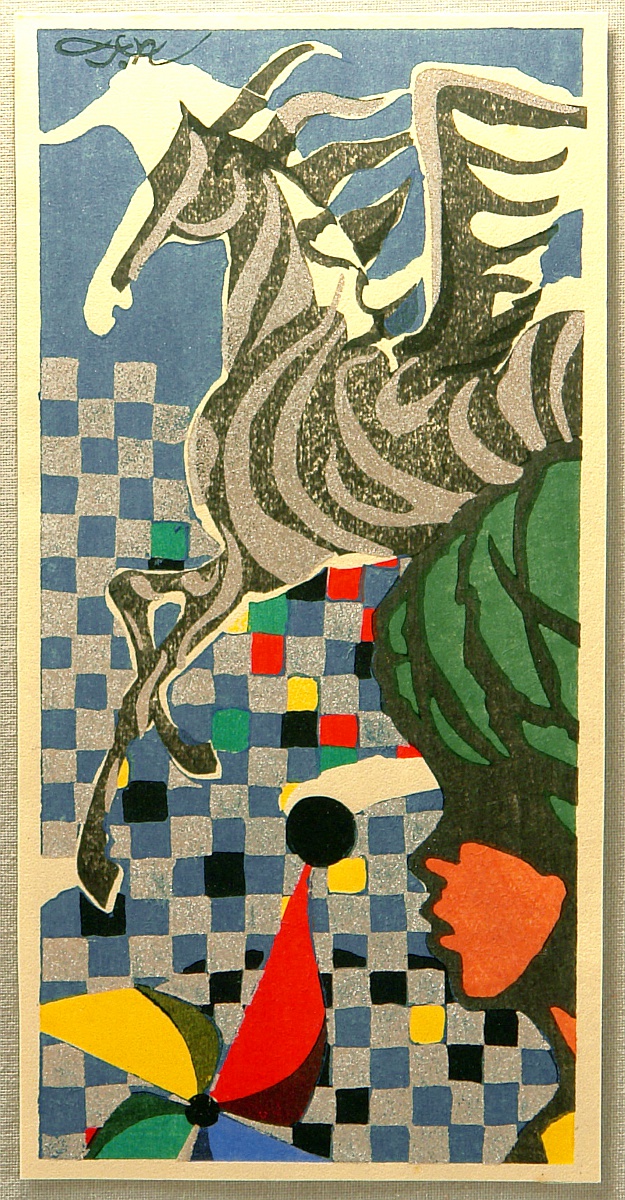The painting is a mixed media artwork in portrait orientation, featuring a captivating blend of elements. Dominating the top half of the canvas is a Pegasus-like horse, reminiscent of a zebra with its gray and dark gray stripes. This mythical creature, with its stringy mane blowing in the wind and delicate wings outstretched, appears to gallop towards the left. Below the Pegasus, in the bottom right corner, is a side profile of a human face, distinct with an orange-brown complexion and adorned with a vibrant green turban, gazing to the left.

The background of the painting is comprised of a detailed checkered pattern in shades of gray and blue, interspersed with colorful squares in red, green, yellow, and black. Adding a playful touch to the composition, a multicolored pinwheel with red, blue, green, and yellow blades occupies the bottom left corner. Encasing the entire scene is a pristine white border, followed by a secondary gray one, drawing the eye towards the artwork's vibrant core. In the top left corner, a signature in cursive green paint subtly claims the artist's credit.